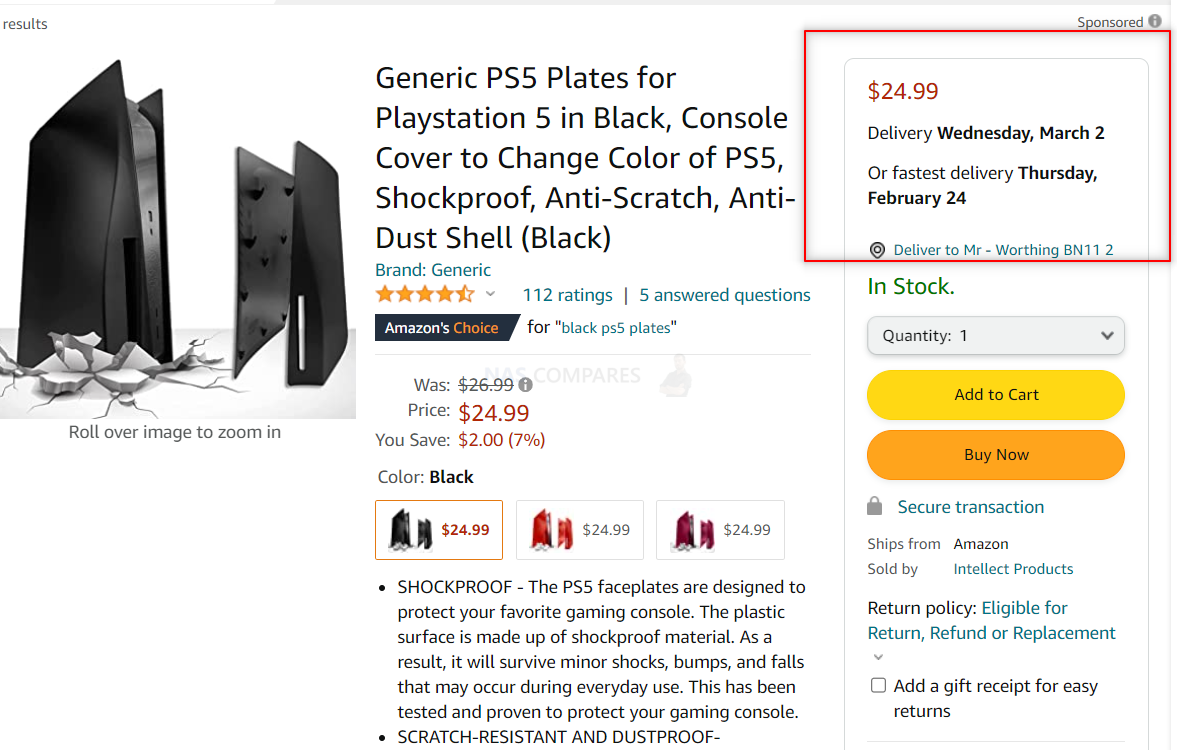This image, taken from an Amazon product listing, primarily features a PlayStation 5 console on the left, accompanied by replacement faceplates in a sleek, matte black color. To the right, the listing advertises these generic PS5 black faceplates, emphasizing their shockproof, anti-scratch, and anti-dust properties, marketed as "shale black." The brand is listed as "Generic," and the price is prominently displayed at $24.99, reduced from $26.99, with delivery options ranging from Wednesday, March 2nd, to an expedited date of Thursday, February 24th. The product's availability is highlighted with an "In Stock" notice and an "Amazon Choice" badge on the left. Additionally, the listing includes three color options at the same price point: the featured black, a reddish-orange, and a burgundy hue. Further details reiterate the faceplates' durability, underscoring their protective features.